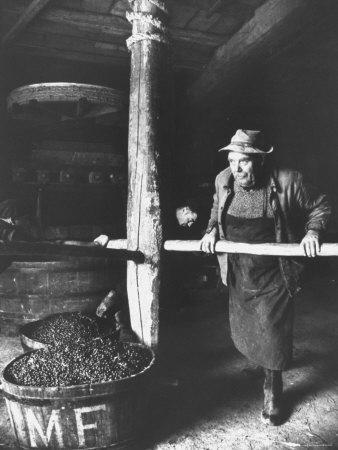In this old black-and-white photograph, two men are depicted in what appears to be a cellar, possibly used for milling or wine pressing. One man is prominently featured, wearing a brimmed hat, an open button-down shirt, a long apron, a sweater, and work boots. He is operating a large grinder or millstone setup that dominates the room. The grinder features a tall vertical post with a horizontal rod extension, which the man is seen pushing to turn the millstone. There are two buckets on the floor near the rod's base, seemingly filled with dark-colored items that might be grapes, small grains, or other produce. These elements suggest the photo captures a scene of traditional milling or pressing, with another man visible in the background holding the opposite side of the pole and assisting with the operation. The attire of the men, including the jackets, indicates that the environment is likely cool.